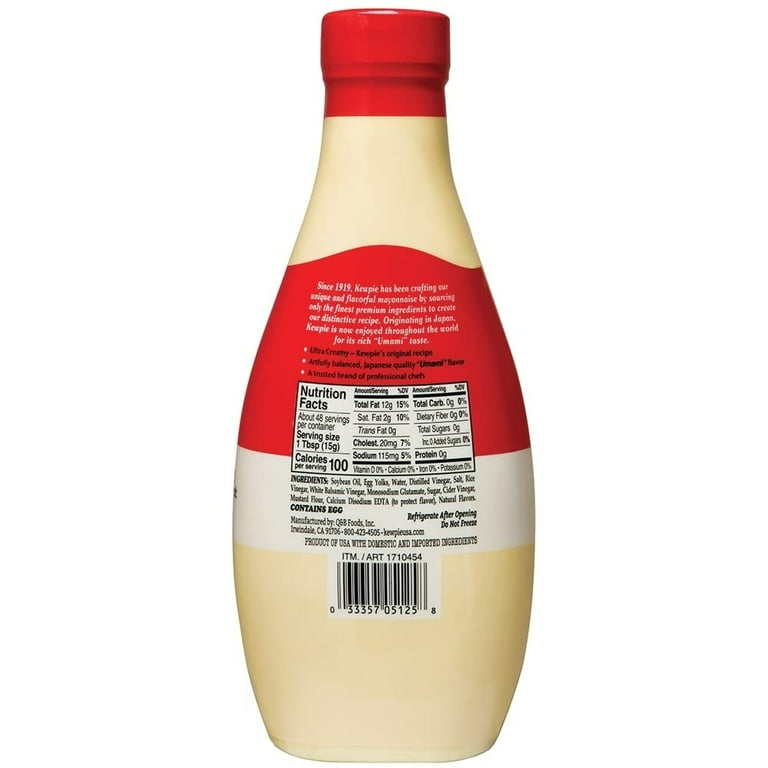The image depicts a Kewpie brand mayonnaise bottle against a white background. The bottle has a unique shape, tapering from a wider base and middle to a narrower top, reminiscent of a vase. The top features a sealed red circular cap, transitioning to a cream-colored section and then a prominent red label. This label includes white and black text detailing the product's origins, nutritional facts (100 calories, 10 grams of total fat, 20 milligrams of cholesterol), and various nutrients like sodium, total carbs, and protein. Additionally, the label specifies that it contains eggs, accompanied by further product details. Beneath the label sits a standard barcode on a white rectangle, while the bottom section of the bottle is cream-colored, suggesting a clear plastic showing the mayonnaise inside. The text highlights Kewpie's long history of crafting mayonnaise since 1919, emphasizing its unique and umami-rich taste derived from premium ingredients.